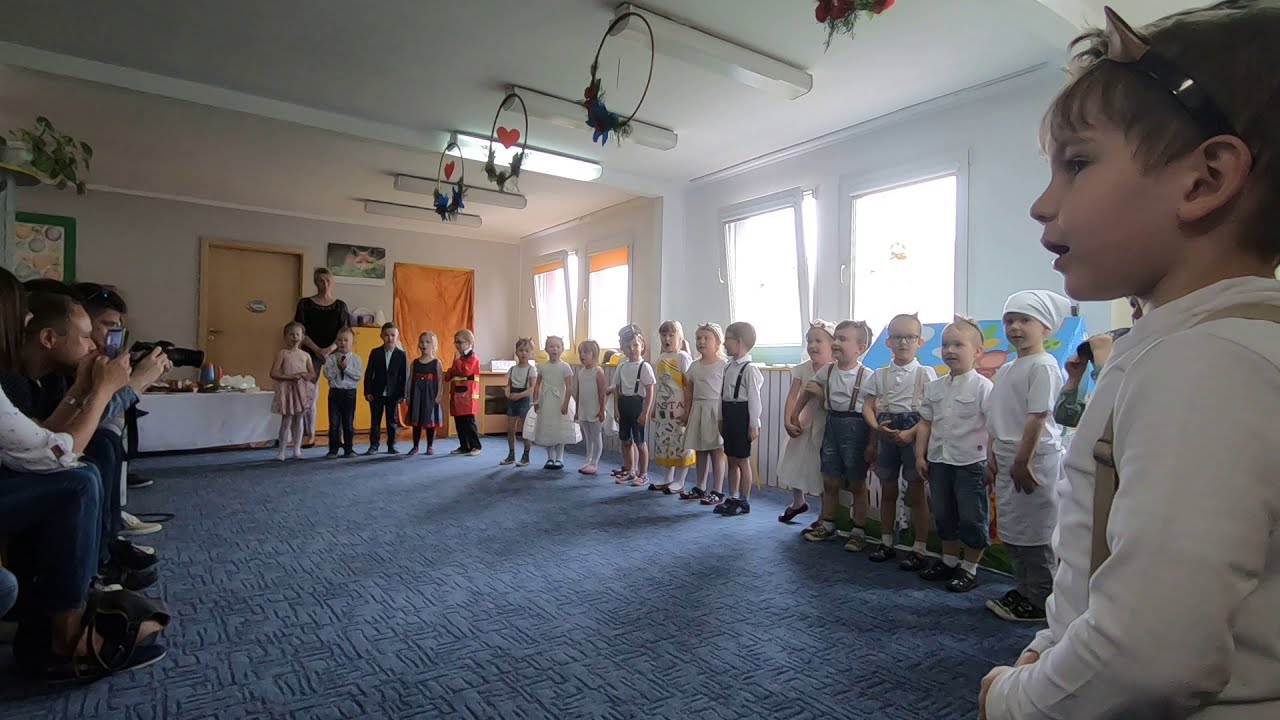The image captures a scene inside what appears to be an elementary school or kindergarten room, featuring a group of young children involved in a recital or play. The children, outfitted in various costumes including superheroes, tuxedos, chefs, and traditional attire with suspenders and bandanas, are lined up and forming a loose semicircle. They are standing on a blue carpet that has distinct patterns, resembling a hieroglyph design, which adds to the character of the room. On the left side, a cluster of parents can be seen seated in chairs, some actively taking pictures or recording the event on their cameras and cell phones. Behind the children, sunlight filters through several windows, illuminating the space. Decorative elements such as hanging hoops with hearts and wreaths adorn the ceiling. In the background, to the left of the children, a teacher or guide stands near a brown door, overseeing the activity. The overall ambiance suggests a festive or performance-related event, possibly a play, Halloween party, or singing recital, with the children joyfully participating in front of their proud families.